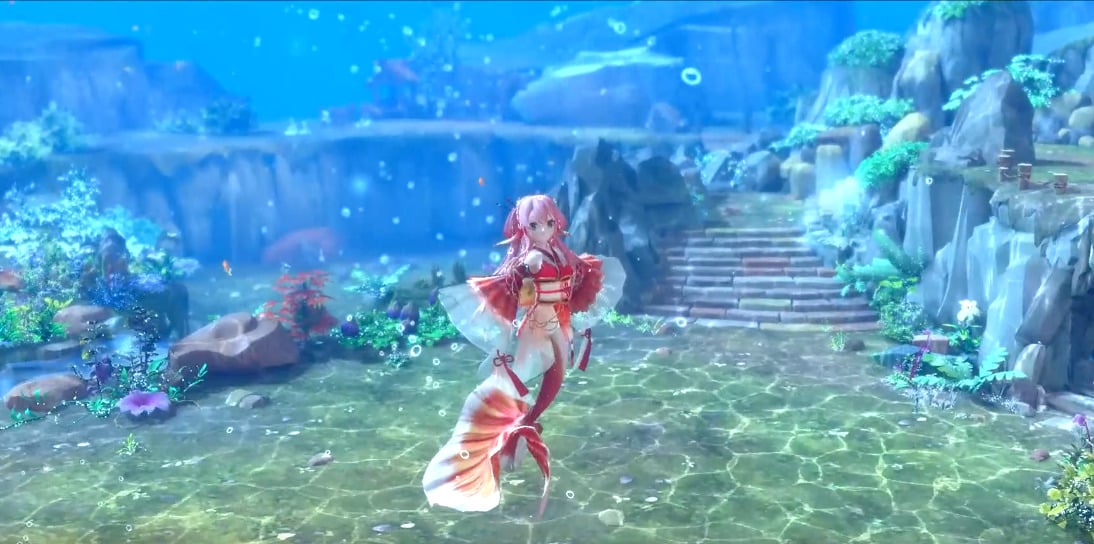In this vibrant underwater scene from a digital graphic, likely an animated movie or video game, a central female character stands out. The image features a mermaid with stunning pink hair and a flowing reddish-pink tail adorned with white accents. She is floating above a greenish stone floor, her arms gracefully spread out to her sides, wearing a red and white, possibly translucent dress. Behind her, stone steps ascend to a platform area, framed by taller, blue rocks with patches of green algae or moss. The background showcases additional cliff-like formations, accentuated by numerous floating bubbles, emphasizing the underwater setting. The overall atmosphere is beautifully detailed, with shades of blue, purple, and green adding to the enchanting, serene scene.